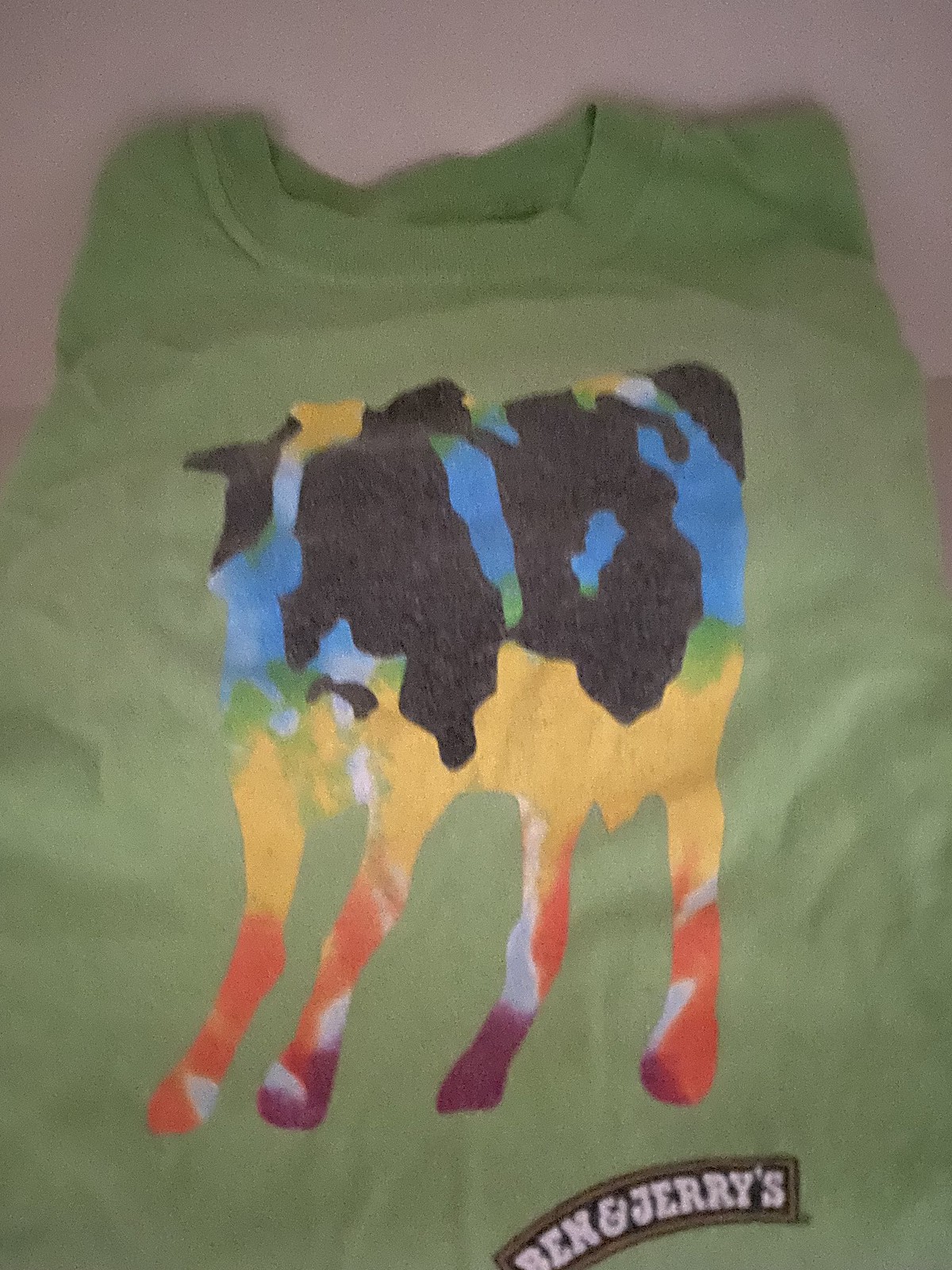The image showcases a green t-shirt from Ben & Jerry's, with a distinctive and vibrant design. Dominating the front of the shirt is a large, multicolored artistic rendering of a cow. The cow features a mosaic of colors including black, blue, green, yellow, orange, red, burgundy, and white, creating a dynamic and somewhat abstract visual, almost reminiscent of a globe's patchwork. The cow's hooves are notably colorful, with two in burgundy and two in orange. Behind the cow, the background is green, suggesting grass. At the bottom right of the shirt, there's a small Ben & Jerry's logo in white text on a black, curved rectangular banner. The sleeves of the t-shirt are not visible, as they appear to be folded underneath. The shirt is laid on a cream-colored surface, and the overall image is slightly blurry.